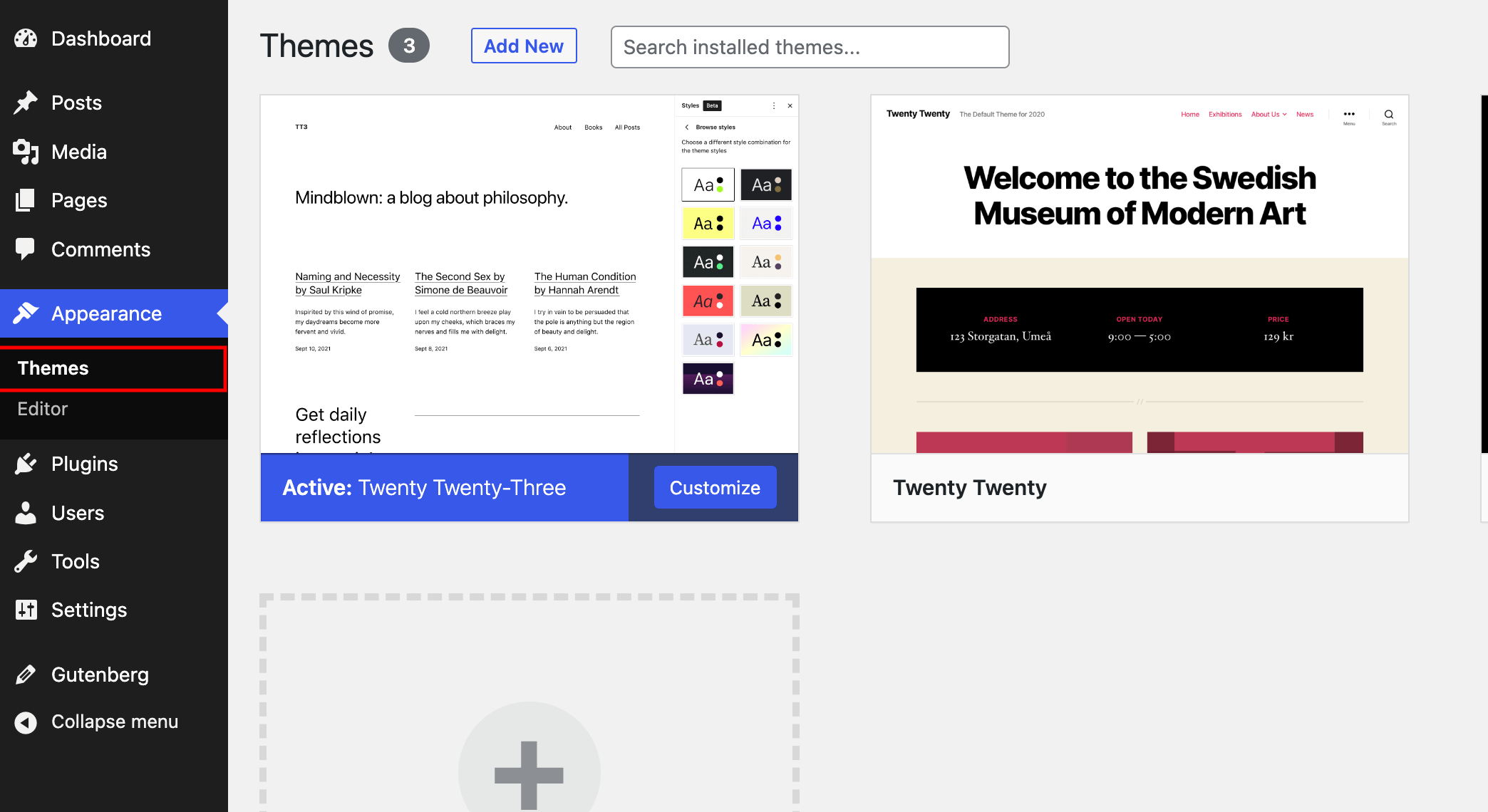The image showcases a thematic interface of a web application. On the far left, a vertical black navigation strip is prominently displayed against a black border. It includes various menu options such as Dashboard, Posts, Media, Pages, Comments, Appearance, Themes, Editor, Plugins, Users, Tools, Settings, Gutenberg, and Collapse Menu.

To the right of this strip, a segment of the webpage highlights the "Themes" section. A grey circle with a white number three is visible on the left side of this section. The "Themes" tab is distinctly marked with a red box, indicating it is the active tab, while the other tabs remain black. The active theme appearance tab itself is noted in blue.

Below the main heading that reads "Themes," additional options such as "Free," "Add New," and "Search Installed Themes" are present. The page also features several blog titles, including "Mind Blown: A Blog About Philosophy," "Naming and Necessity by Sol Kripke," "The Second Sex by Seymour de Beauvoir," and "The Human Condition by Hannah Arendt."

On the right side of the interface, there are numerous sample style sets available for browsing. These feature various font sizes marked by uppercase 'A' and lowercase 'a', along with two circles indicating different color options and varied background colors.

Overall, the detailed layout of the thematic interface and the careful organization of options allow for a user-friendly and visually distinct experience.